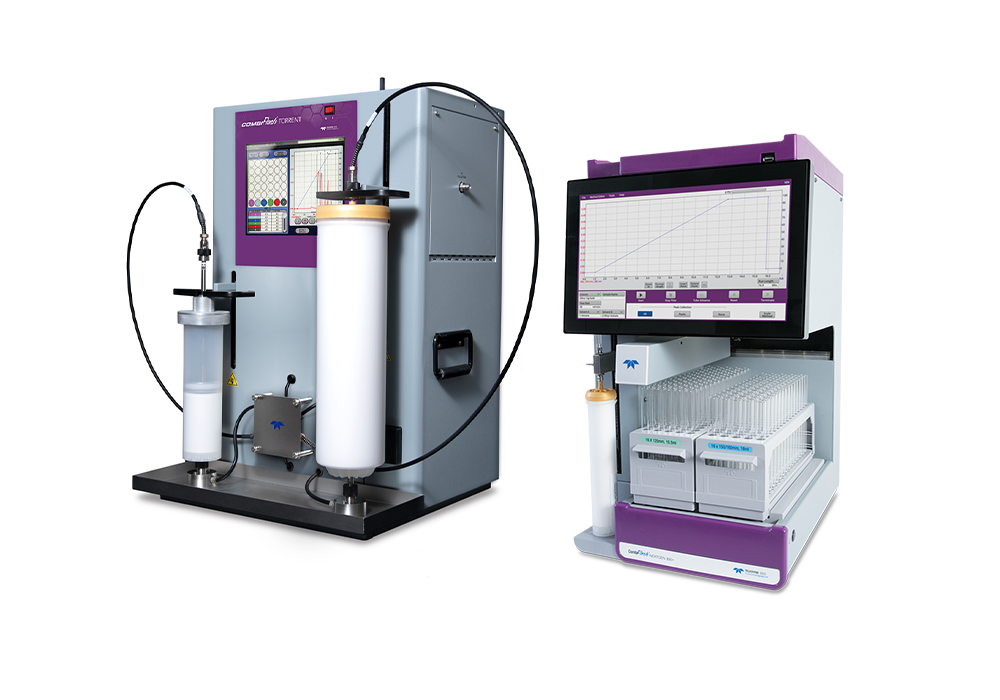In this image, we see three large machines with a white background, arranged from left to right in descending order of height. On the far left is the tallest machine, which is gray with purple accents. It features a smaller screen displaying a line graph, and has large cylinders attached to black tubes. In the middle stands a slightly smaller gray machine, also with a screen showing data in the form of graphs. This machine is equipped with glass tubes and metal cylinders within its structure. The machine on the far right is the smallest. It is gray with purple accents, and has a large screen displaying information, with additional tubes or glass discs held in a white basket below it. This equipment appears to be medical or scientific measuring devices, reminiscent of ATMs in size, but with specialized features like data screens, tubing, and glass components.